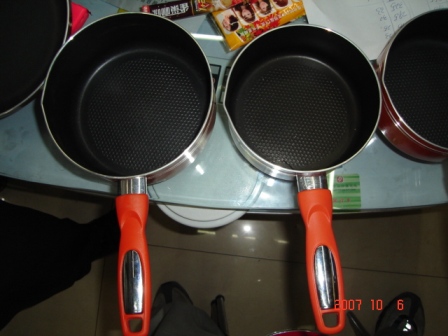The image is a low-resolution, color photo taken indoors from a bird's eye view, depicting a set of four cooking pots resting on a countertop or stove. The image is timestamped "2007-10-6" in the bottom right corner. Of the four pots, two are fully visible, with vibrant orange plastic handles covering their stainless steel grips. Another pot is partially visible on the right, showing about half of it, while a third pot on the left shows about a third. These round saucepans and a frying pan feature black, likely non-stick interiors, and one of them has a spouted tip. The largest pot is slightly bigger than the ones on the right. Additional details include the feet of two individuals in the lower part of the photo: one in black pants and shoes, and another in gray pants. Behind the pans, a Hershey's Special Dark Chocolate bar and another indistinguishable wrapped item are visible on the countertop.